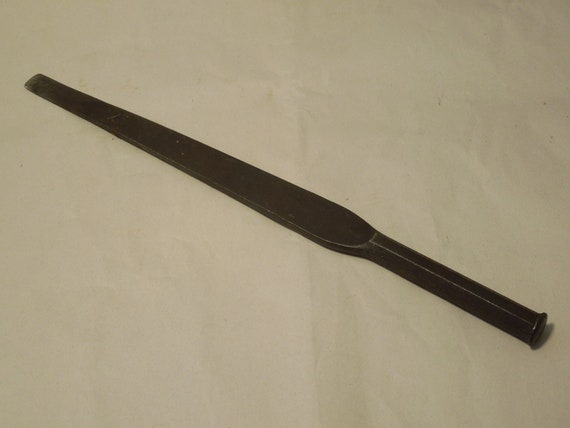The photograph showcases a mysterious black object placed on a light-colored surface, which could either be off-white, very light brown, or light gray, resembling wood, linoleum, or possibly paper. The lighting is not ideal, making it difficult to definitively ascertain the object's identity. The object has a prominent circular, flared end that transitions into a square section before flattening out into a shape reminiscent of a spatula or paddle. This section extends into a flat, elongated body that appears narrow yet broad enough, giving it a somewhat chisel-like or scraper-like appearance. The object is approximately a foot or more in length, with its thicker end potentially designed to be held or struck. The surface detail is limited, providing no additional clues as to the object's specific purpose, whether it be a kitchen implement, a musical instrument, or a specialized tool. Overall, its unique shape and ambiguous function add to its enigmatic presence in the photo.